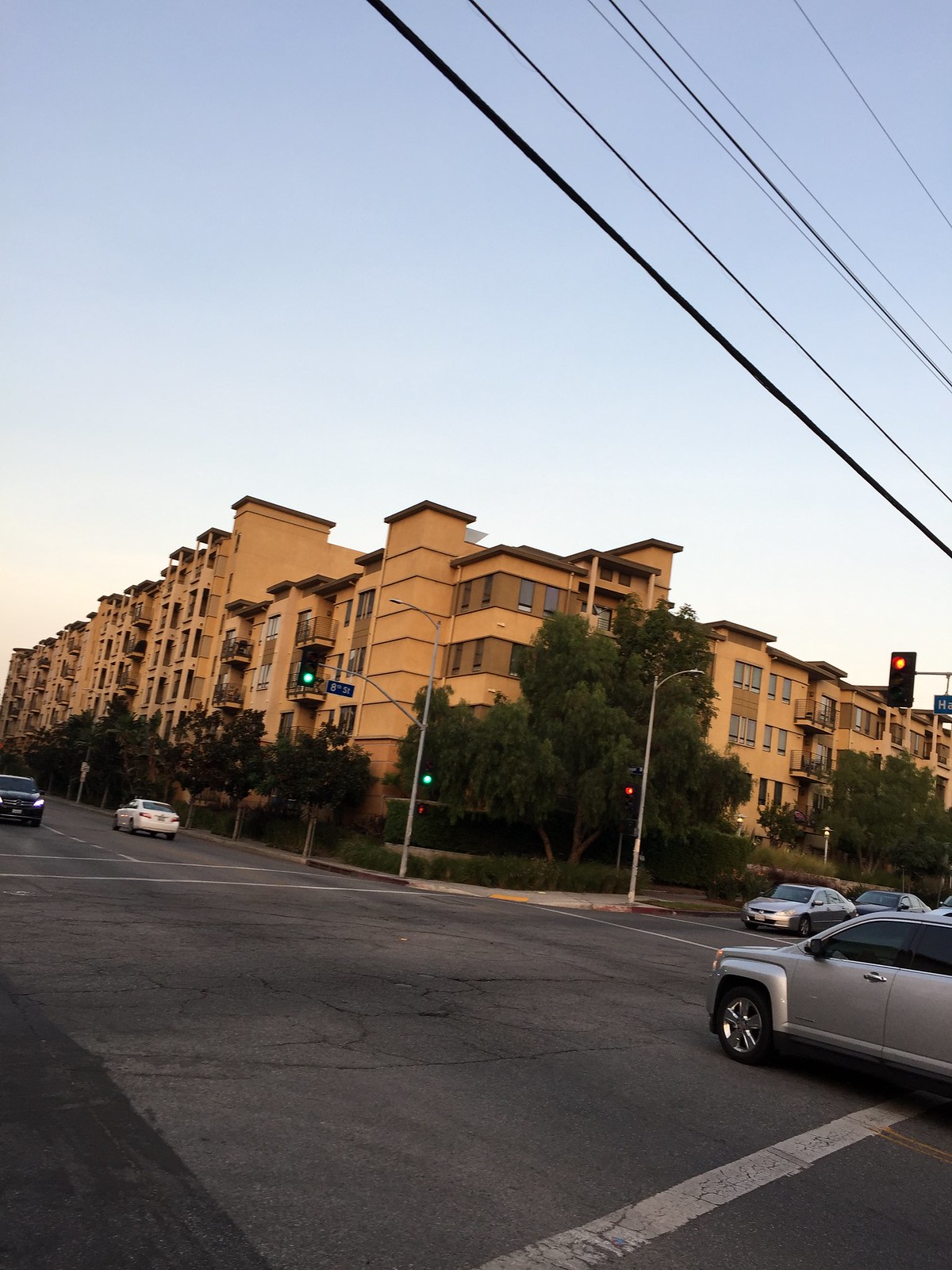This photograph captures a busy urban intersection featuring distinct crosswalk lines and streetlights. The view is diagonally across the crossroads, highlighting the intersection of 8th Street, marked prominently by a street sign. 8th Street, which runs from the lower left to the upper right, currently shows a red traffic light. The intersecting street, which begins with "HA," runs from the lower right to the upper left and has a green traffic light.

On the far right of the image, a silver SUV is seen entering the intersection. Just above it, two cars—one silver and the other appearing black—are stopped at the red light. In the top left corner, a white car is moving away from the intersection, while a black SUV is poised to enter.

A large apartment building dominates the background on the corner. This structure features a medium tan facade with darker brown trim, multiple balconies, and numerous windows. It has a flat roof and is segmented into a lower section about four stories high and a taller section rising to six stories. The building is fronted by green trees and bushes, with a hedgerow separating the sidewalk from the building.